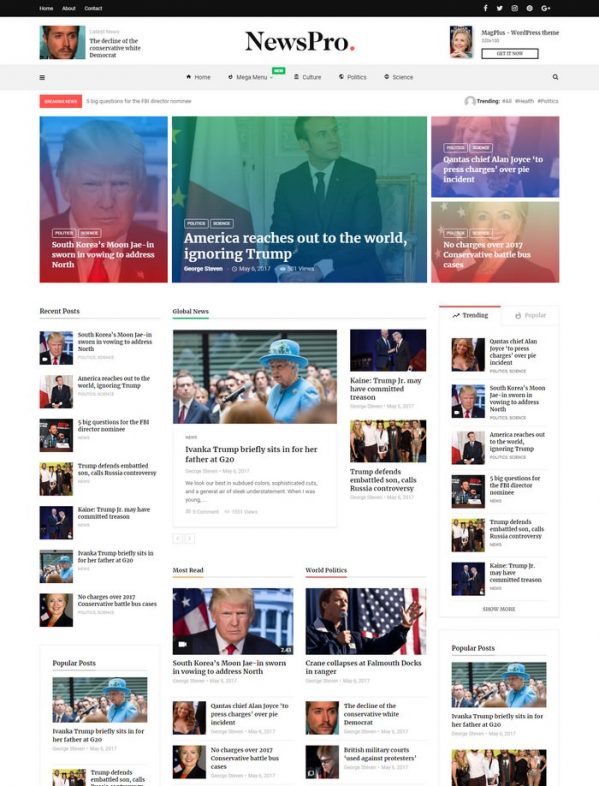Screenshot of a news website with a clean, white background. On the top right corner, there's a logo labeled "News Pro". The layout features a gray search bar with a magnifying glass icon to the right. Below the search bar is a black navigation bar containing links: "Home," "About," and "Contact."

The page displays multiple articles with accompanying images. On the left, there's a headline reading "America Reaches Out to the World, Ignoring Trump" with a picture of former President Trump and another man. Below this, there is an image of a woman followed by another woman, next to the headline "Global News."

Further down is a snippet titled "Ivanka Trump briefly sits in for her father at G20," accompanied by an image of the Queen and another image of Ivanka Trump. The right sidebar contains a section labeled "Popular Posts," listing several articles, reinforcing the "Global News" theme.